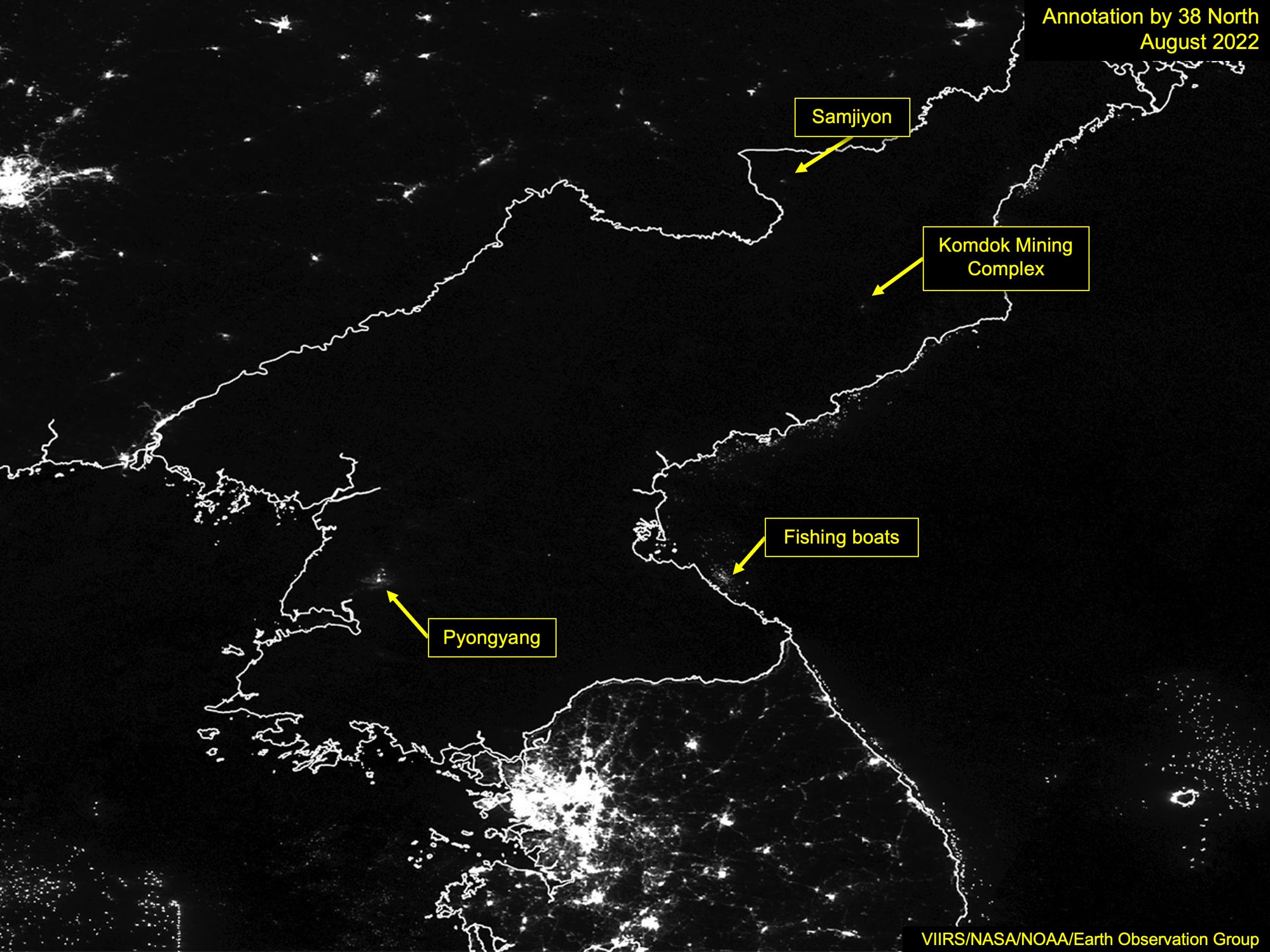This black and white satellite photograph captures a detailed view of North Korea and its surrounding regions, with borders outlined in white. The image prominently features annotations made in August 2022 by 38 North, VIIRS, NASA, NOAA, and the Earth Observation Group, which are noted in the top right and bottom right corners in yellow text. The photograph highlights key areas with yellow arrows and text, showing significant locations such as the Payong, Fishing Boats, Komodo Mining Complex, and Siami Zone. The few illuminated spots in North Korea contrast starkly with the brightly lit areas in South Korea below the border and China above. This digitally created map effectively displays the geographic and infrastructural elements, with a focus on water and land areas, and the distribution of light emissions in the region.